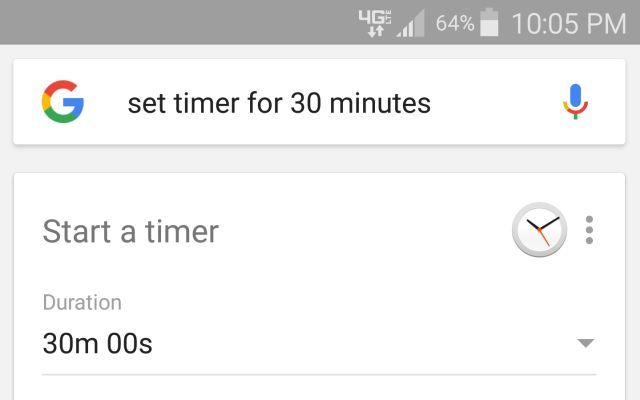A detailed screenshot of a smartphone interface displaying various status indicators and a timer setup. The top gray status bar shows a '4G' signal indicator, a battery level at 64%, and the current time, 10:05 PM. Below, in a white section with a gray background, there's a Google app icon beside the text "Set timer for 30 minutes," and a microphone icon on the far right, indicating a voice command preference. The next segment is a larger white box featuring a timer setup interface. It displays the prompt "Start a timer" alongside an illustration of an old-fashioned clock with hour and minute hands. On the right-hand side, there's a vertical ellipsis (three vertical dots) menu. Further below, it details the timer's duration set to "30m 00s" (30 minutes and 0 seconds) with a downward-pointing arrow on the right side. The entire interface is showcased on a clean white background.